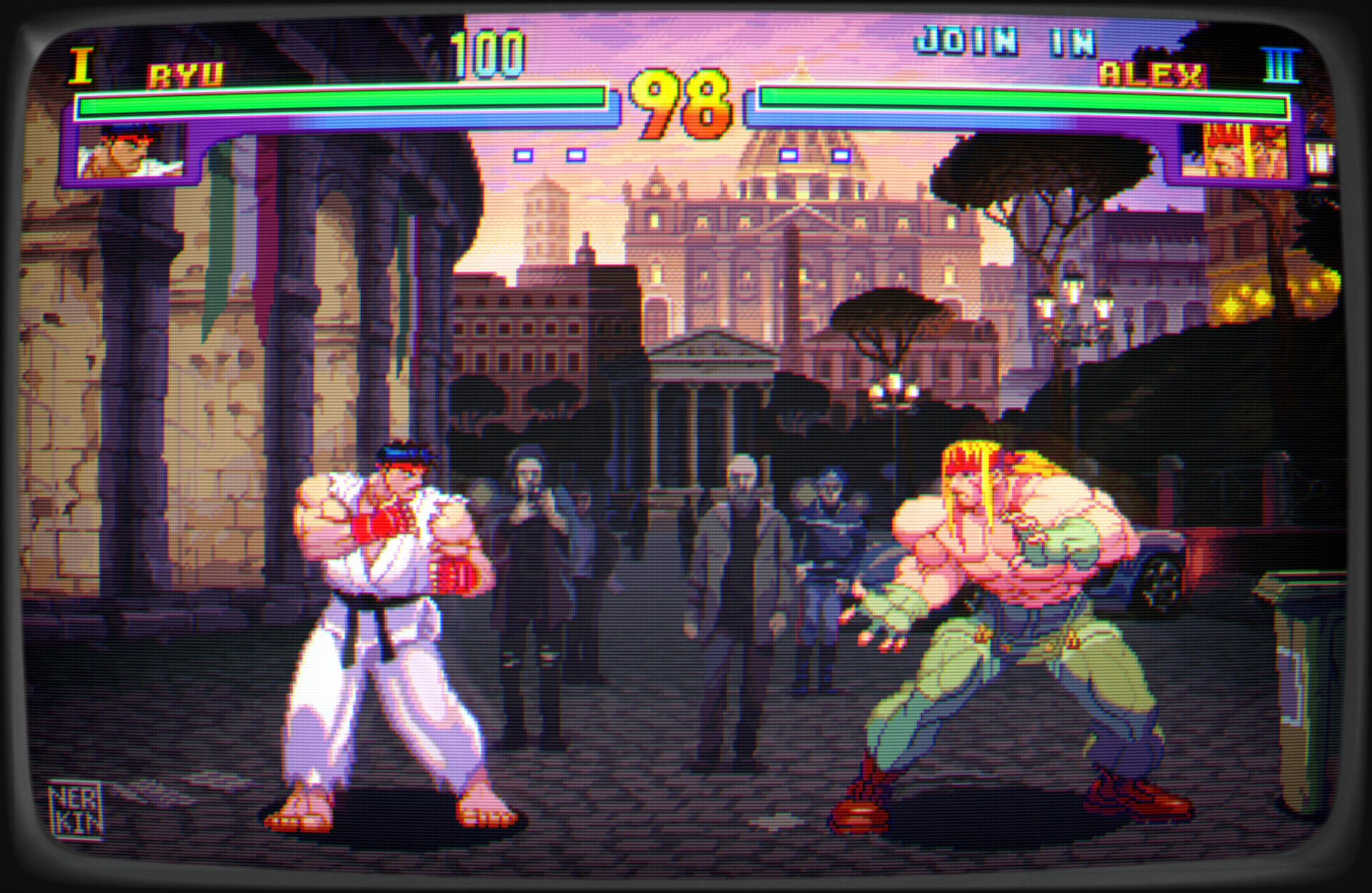This image is a detailed screenshot from the classic video game Street Fighter. It captures a moment just before the fight begins between two well-known characters, Ryu and Alex. The scene is set on a cobblestone street in what seems to be an Italian city, evidenced by Italian flags and architectural elements in the background. Ryu, positioned on the left, is dressed in a traditional white gi with a black belt, red gloves, and a blue headband. His opponent, Alex, stands on the right, muscular and shirtless, adorned with green pants, a red bandana, and red shoes. Both characters have full green health meters above them, marked with '100' for Ryu and an additional '98' in yellow and red. The background teems with cartoon-like spectators, presumably computer-generated, lined up and attentively watching the impending clash. In the lower part of the screen, there is also a white box with text that partially reads "join in," indicating that the game is ready for the next player.